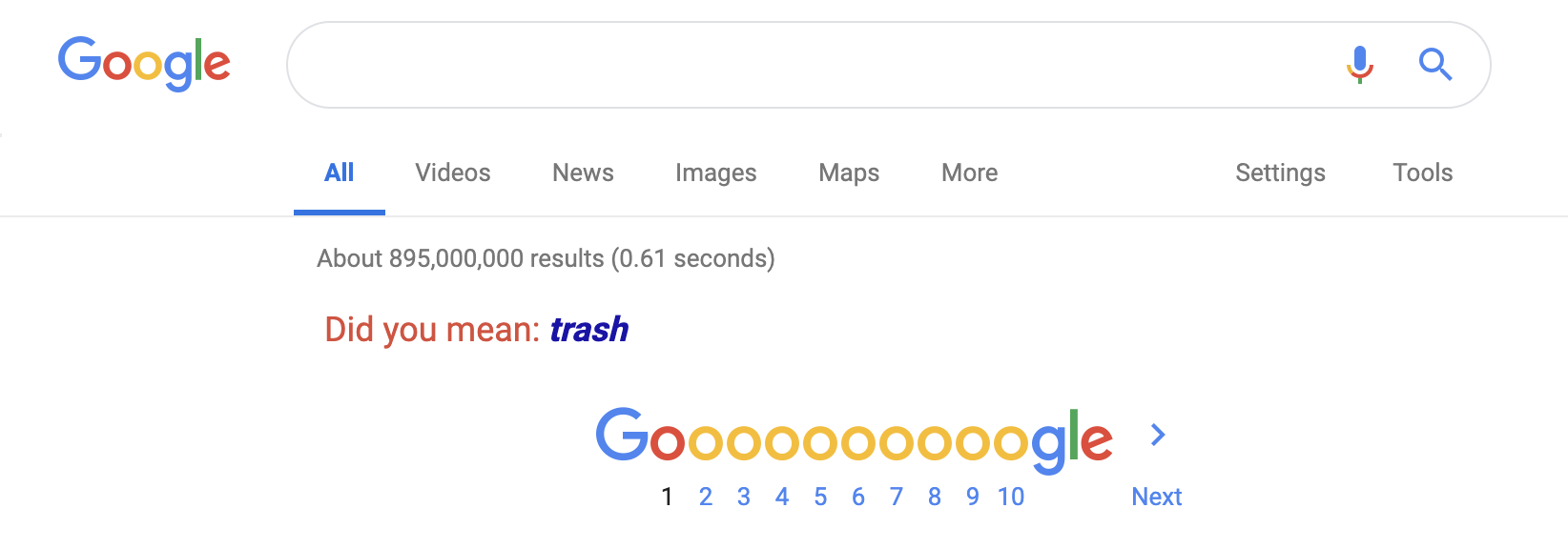The image features a Google search results page with various elements. In the top-left corner, the familiar Google logo is present, followed by an oblong search bar outlined in gray. Inside the search bar, the Google microphone icon is situated, symbolizing the voice search function, and on the far right end of the bar, a blue magnifying glass icon is located, indicating the search button.

Below the search bar are eight navigational options. The first option, labeled "All," is highlighted in blue letters and underlined with a blue bar. The subsequent options are "Videos," "News," "Images," "Maps," and "More," all written in black text. Additionally, there is a space followed by "Settings" and "Tools" on the right.

A gray bar spans horizontally across the screen, beneath which the search results information is displayed: "About 895,000,000 results (0.61 seconds)." Below this line, in red text, is "Did you mean:" signaling a search correction suggestion.

The suggested term "trash" is prominently bolded and italicized in navy letters. Directly underneath, there is a stylized Google logo followed by an arrow pointing to the right. This logo is creatively depicted with a capital "G" in blue, followed by a lowercase "o" in red, nine lowercase "o"s in yellow, a lowercase "g" in blue, a lowercase "l" in green, and finishing with a lowercase "e" in red.